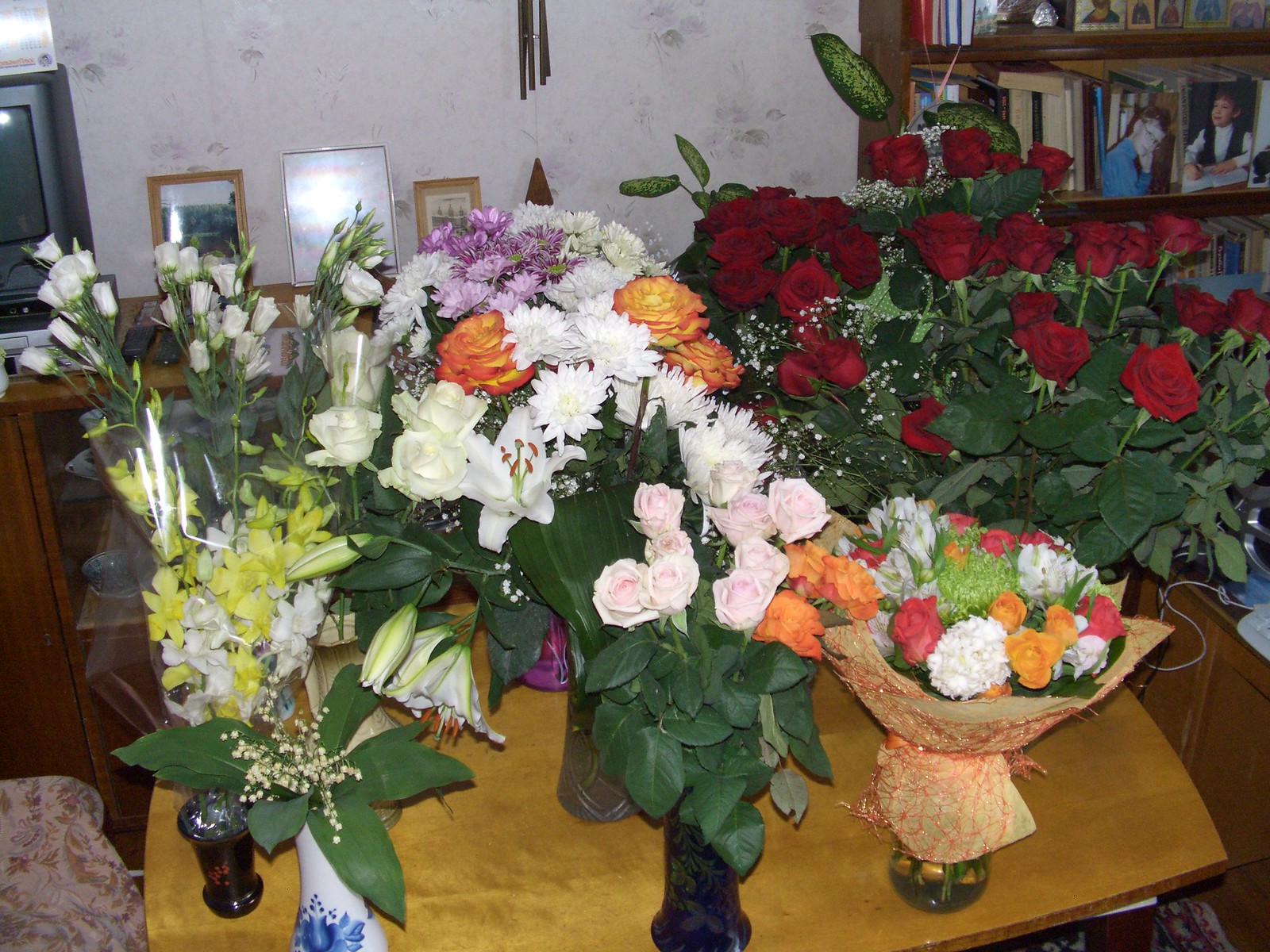The photograph captures an intimate glimpse into a home setting, featuring a table laden with a diverse array of flower bouquets. The table, draped in brown paper, hosts a stunning variety of flowers including red, pink, and orange roses, white lilies, carnations, and mixed bouquets all accentuated by lush greenery. The flowers are arranged in an assortment of vases, ranging from elegant blue and white porcelain and clear glass to subtle black vessels. To the left, a vintage television set with a VCR is positioned above a dark brown glass-fronted cabinet displaying blue and white china. The bottom left corner hints at a floral-patterned piece of furniture. In the background, the pale pink wallpaper with a delicate floral design adds a charming touch, while the top right corner reveals a wooden bookcase populated with books and framed family photographs, and a wind chime hanging against the wall completes the cozy domestic scene.